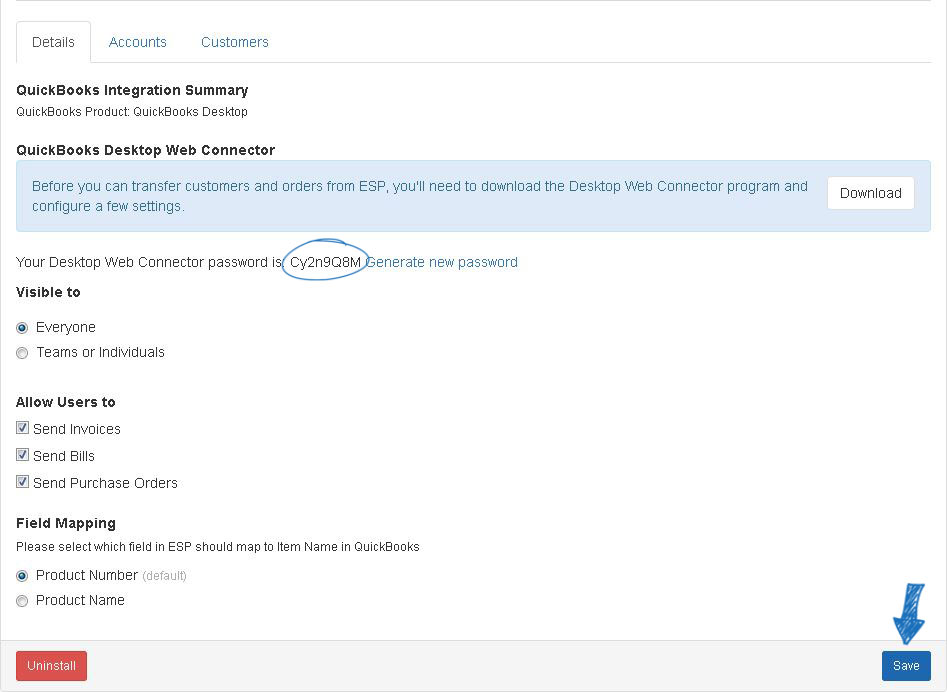The image is a screenshot from a website detailing a section titled "QuickBooks Integration Summary." At the top of the page, there are three tabs: "Details," "Accounts," and "Summary," with the "Details" tab being currently selected. The content under this tab provides instructions for integrating QuickBooks with another system, specifically indicating the QuickBooks Desktop and QuickBooks Desktop Web Connector products. The text instructs that before transferring customers and orders from ESP, users need to download the Desktop Web Connector program and configure a few settings. A prominent "Download" button is situated on the right side of the page.